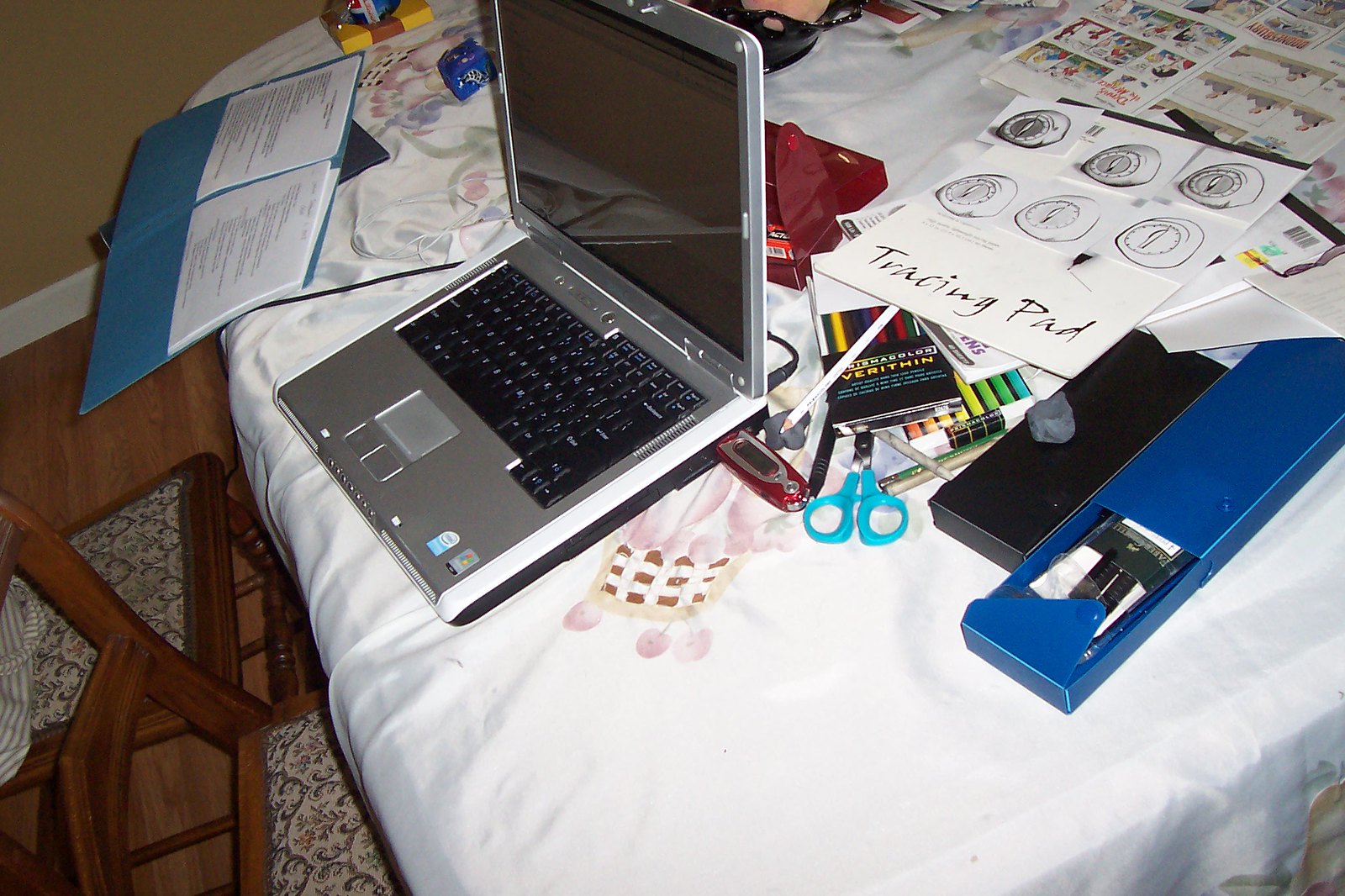The image depicts a cluttered table, signifying a space used for creative work, possibly drawing or tracing. Centered prominently is an old, silver laptop made of plastic, suggesting the photo may date back to the mid-2000s or 2010s. The laptop is open, displaying its black keyboard and screen, with a red USB stick inserted into it. 

Surrounding the laptop, the table is strewn with various stationery items, including blue-handled scissors, standard pencils, and colored pencils, the latter partially hidden under a sheet labeled "tracing pad." To the left of the laptop lies an open blue folder, bulging with paperwork in both its left and right pockets. 

Additionally, a blue box and a black box are situated on the table, their contents unknown. Atop the black box, there is a broken eraser piece. The setting is completed with a white tablecloth covering the table and a wooden chair nearby, suggesting a casual yet industrious atmosphere. This detailed scene provides a glimpse into a workspace dedicated to artistic or technical tasks.